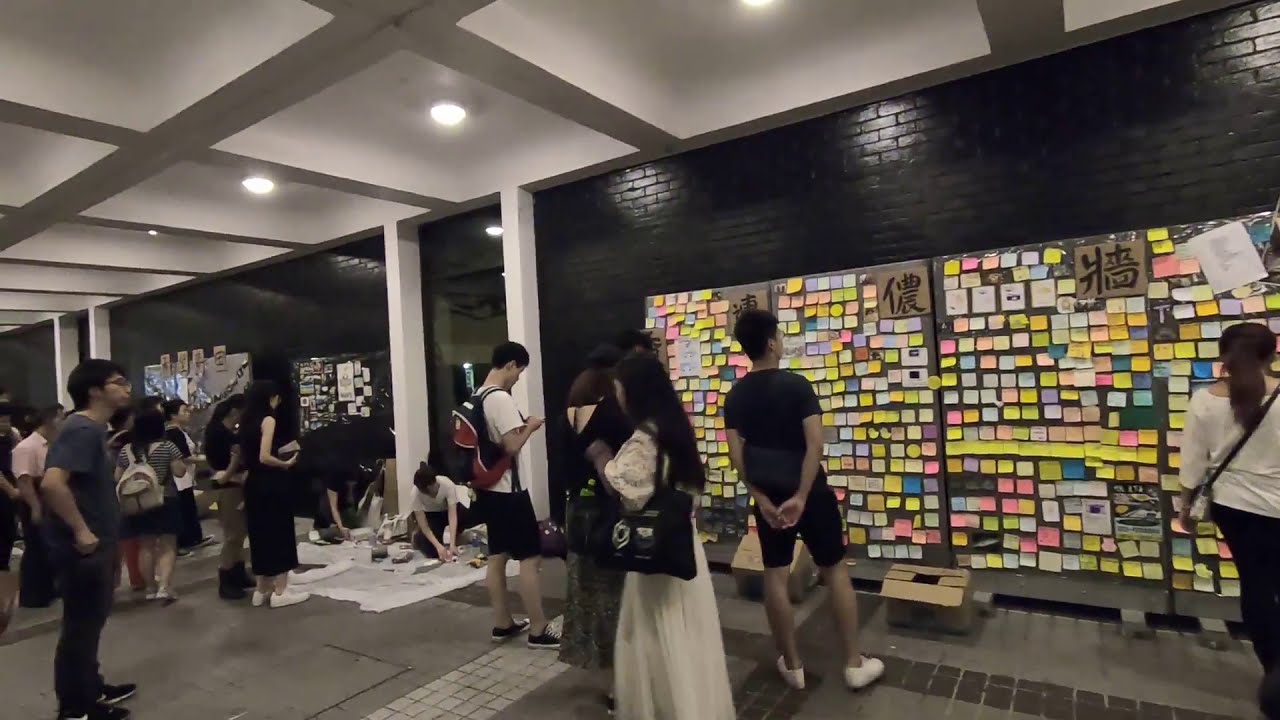Inside a modern building, possibly in an Asian community or country, a group of young adults, likely in their 20s, are engaged in viewing various exhibits mounted on black brick walls. The building features a ceiling of white square panels, each housing a light, and the floor is covered in gray and brown tiles. The walls include open doorways or windows framed in white. 

To the right, three large panels with a gray background are completely covered in multicolored post-it notes, and several people are clustered in front of these displays, intently examining them. Among the post-it notes, there is a noticeable brown square in the top right corner with Chinese characters. Throughout the room, other displays are also mounted on the walls with more people observing, although these displays are not clearly visible. 

Additionally, in the central part of the room, a group appears to be actively working on a project atop a large drop cloth on the floor, using paint or other media. Some of the people in the room have backpacks and purses, adding to the impression of a casual, collaborative atmosphere possibly linked to an educational or studio setting. The environment suggests a dynamic, creative space where both the viewing and creation of art or information are taking place.